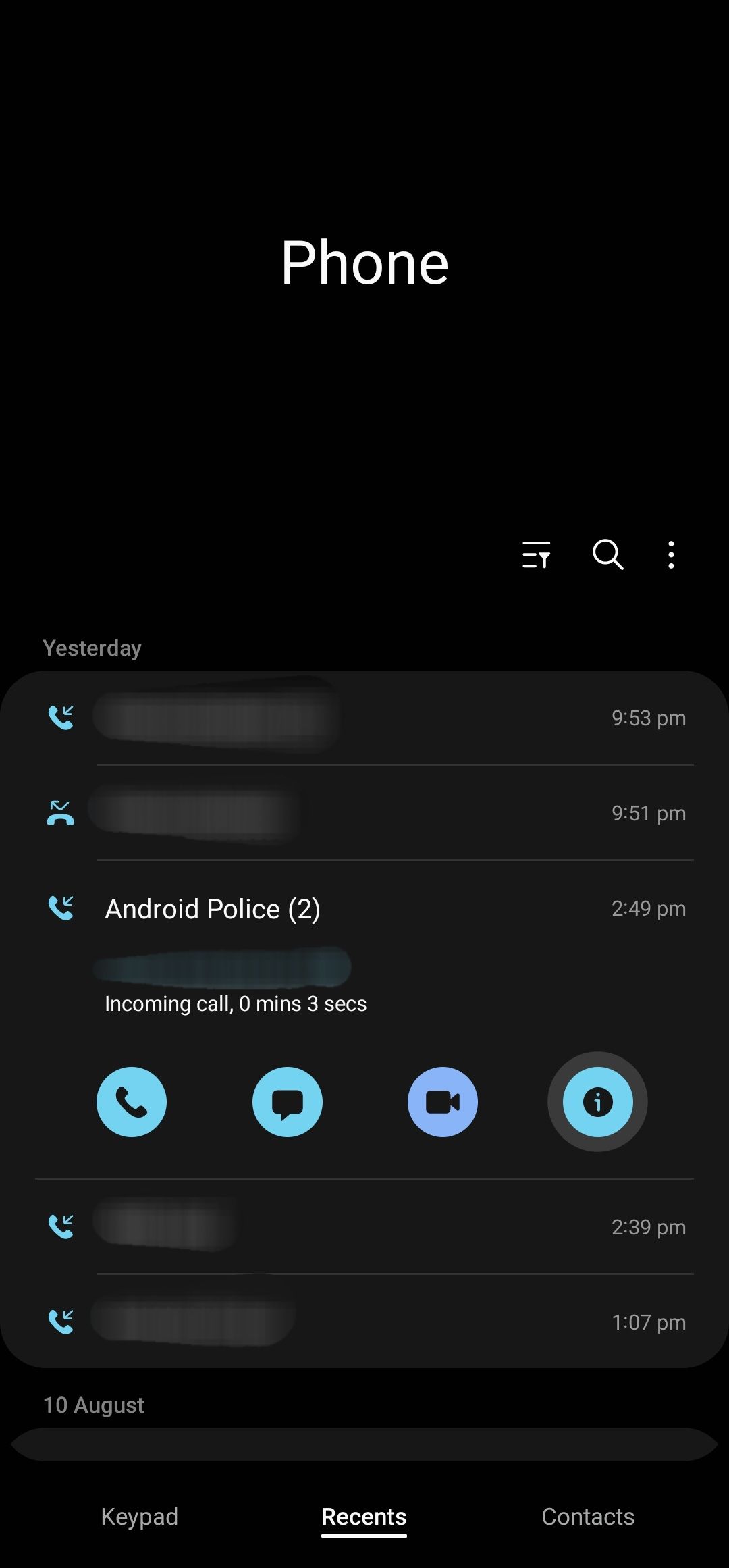This vertical rectangular image is a screenshot from a smartphone, displaying a call log against a completely black background. At the top center of the screen, the word "Phone" is clearly spelled out in white text. 

Below this top section, a chronological call list begins with a heading that reads "Yesterday". The first entry is an incoming call at 9:53 p.m., followed by a missed call at 9:51 p.m.; the details of these entries are blurred for privacy. Next, there is an incoming call from "Android Police" with a notation "(2)" at 2:49 p.m., denoting that there were two recent interactions. This entry notes the call was incoming and lasted zero minutes and three seconds, but part of this information is also blurred.

In the middle section of the screen are four distinct blue circular icons. Each icon has a different symbol: a phone, a text box, a video camera, and an eye inside a black circle.

Further down, there are two more blurred call entries: one at 2:39 p.m. and another at 1:07 p.m. The entries marked "10th of August" begin but are cut off by the bottom edge of the screen.

At the very bottom, there is a navigation bar with three options: "Keypad," "Recents," and "Contacts." The "Recents" tab is currently selected.